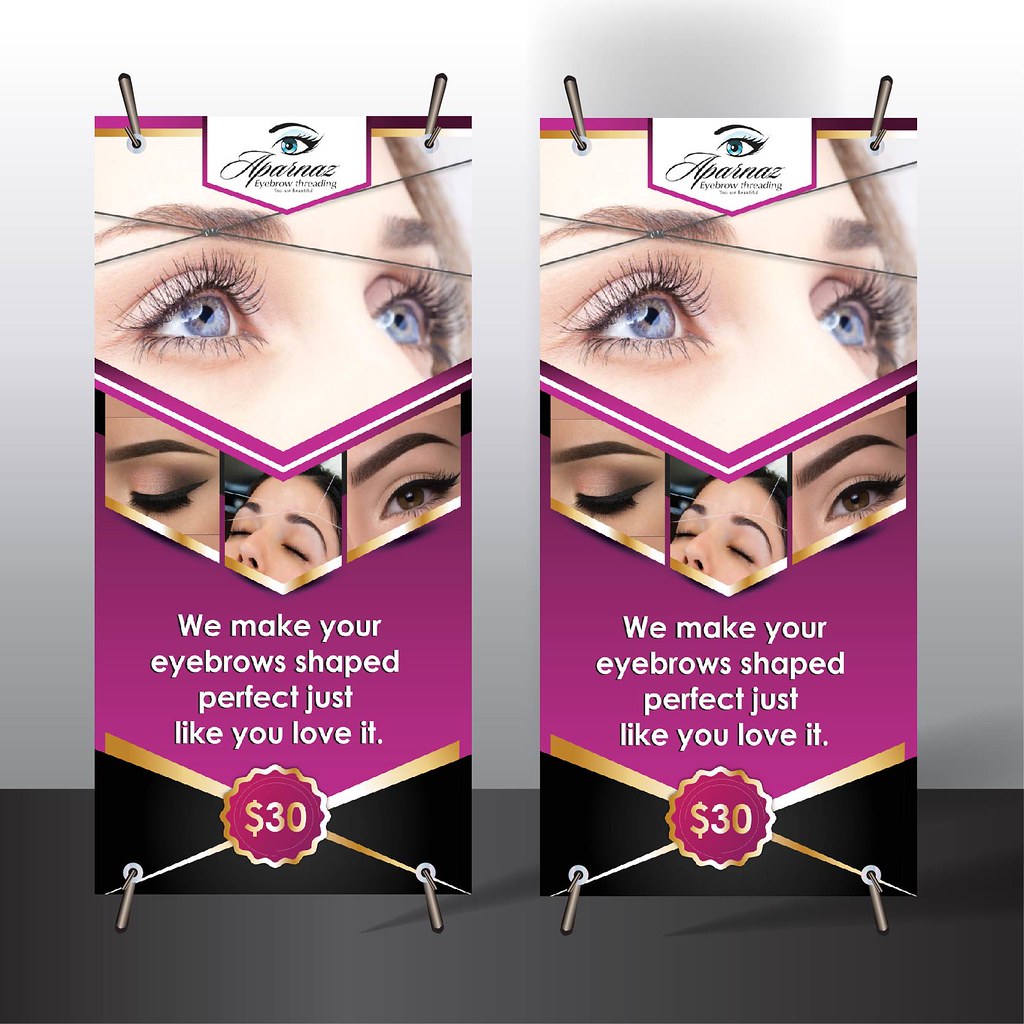In this image, there are two identical stand-up banners placed side by side, each showcasing an advertisement for Aparnaz Eyebrow Threading. At the top of the banners, in stylish cursive text, is the name "Aparnaz," followed by "Eyebrow Threading" in smaller letters below. Below the title, there is a prominent photograph of a woman with blue eyes and white skin, focusing on her eyelashes. Beneath this main image, there are three additional photos: the first is of a closed eye emphasizing the eyebrow and eyelashes, the second shows a woman's face from her forehead to her nose with closed eyes, and the third features a close-up of a single open eye with brown eyes, detailed with winged liner and filled-in brows. Below these images, white text on the banner reads, "We make your eyebrows shaped perfect, just like you love it," followed by a small red star indicating a price of $30. The overall background of the banners appears to be gray.